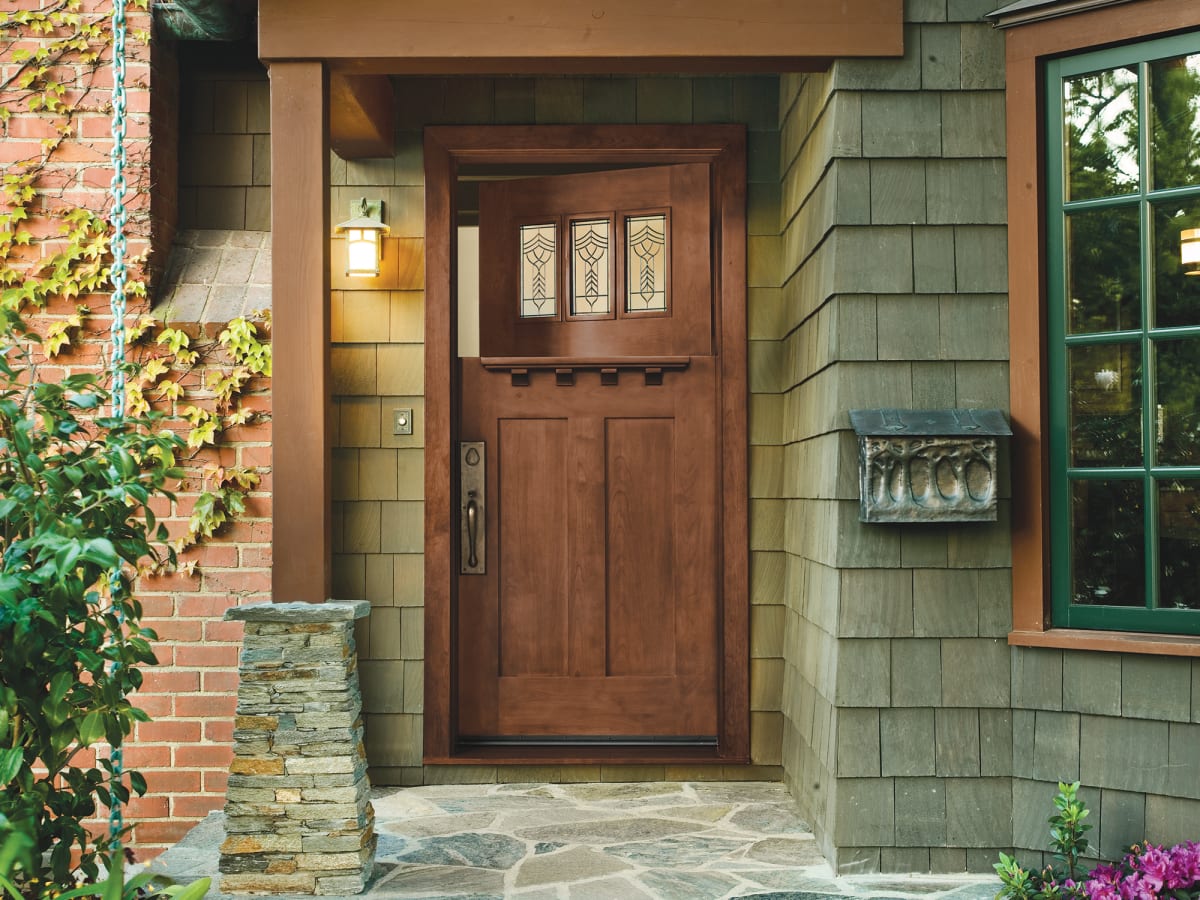This image captures the front porch of a charming home with a distinctive rustic appeal. The exterior of the house combines olive green wooden shingles with patches of red brick to the left of the entrance. A partial wooden pillar with a sturdy stone base stands prominently, supporting the roof and adding to the rustic aesthetic. The patio features large, decorative stone pavers leading up to a dark wooden door, which is uniquely divided into two parts. The lower half of the door is closed, while the upper half, containing three small window panels, is slightly open, allowing for an airy feel and functionality. Beside the door, to the left, a small rectangular light glows warmly, enhancing the welcoming atmosphere. Above this, ivy gracefully climbs the brick wall. To the right side of the door, a metal mailbox with tree-shaped impressions adds a touch of charm. Further right, beneath a window with a dark hunter green frame, a small plant with vibrant pink and purple flowers blooms, completing the quaint and inviting scene.